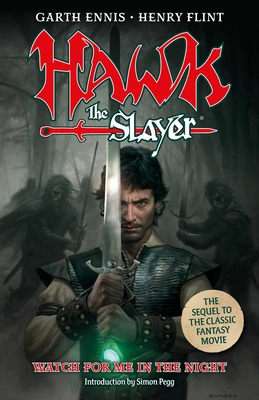The book cover for "Hawk the Slayer" prominently features a central figure, a white male with a wild mane of dark hair and a mustache, looking intensely angry and serious. He is dressed in rugged leather armor designed to offer protection, suggesting a medieval or fantasy setting. His right arm sports a white shirt band and a leather bracelet just before his hand, which grasps a broad sword. The sword, tapering from its guard, bears a glowing green gem at its base. Behind him, shadowy figures holding swords imply looming threats or enemies. 

The title "Hawk" is boldly inscribed in sharp, angular red letters, interconnected in a distinctive style, with "The Slayer" written in white beneath it, placed over the image of a red sword. Above, the names of the authors, Garth Ennis and Henry Flint, are displayed on a dark banner. Below the central figure, green illumination underscores the phrase "Watch for me in the night." An introduction by Simon Pegg is also mentioned.

A tan circle to the right declares in green text, "The sequel to the classic fantasy movie." The overall color palette of the cover is dominated by grays and blacks, enhancing the dramatic and intense visual impact of the scene.